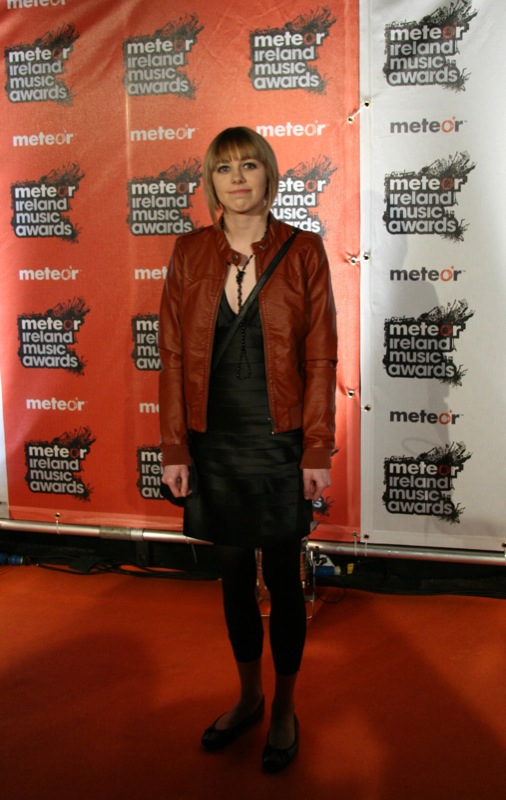In this photograph taken at the Meteor Island (occasionally referred to as Ireland) Music Awards, a young woman, possibly in her early 20s and of Caucasian descent, stands confidently on the red carpet. The portrait-mode image captures her from head to toe, emphasizing her chic and stylish appearance. She has short blonde hair cut into a bob that frames her face delicately, and her light skin tone is complemented by her fashion choices. Her mouth is pursed into a thin red line, giving her a semi-smile, and she is looking slightly upwards and past the photographer.

She is dressed in a striking dark red leather jacket, which she wears over a sleek black ensemble consisting of a dress, leggings, and black slip-on shoes. A small purse is slung across her chest, adding to her fashionable look. The backdrop behind her is divided into two sections, predominantly occupied by banners promoting the event. Most of the backdrop is a bold orange with the logo "Meteor Island Music Awards" repetitively printed, while a portion on the right side features the same logo but on a white background. The vibrant colors of the backdrop—orange and white—contrast sharply with her dark red and black attire, making her the focal point of the photograph.